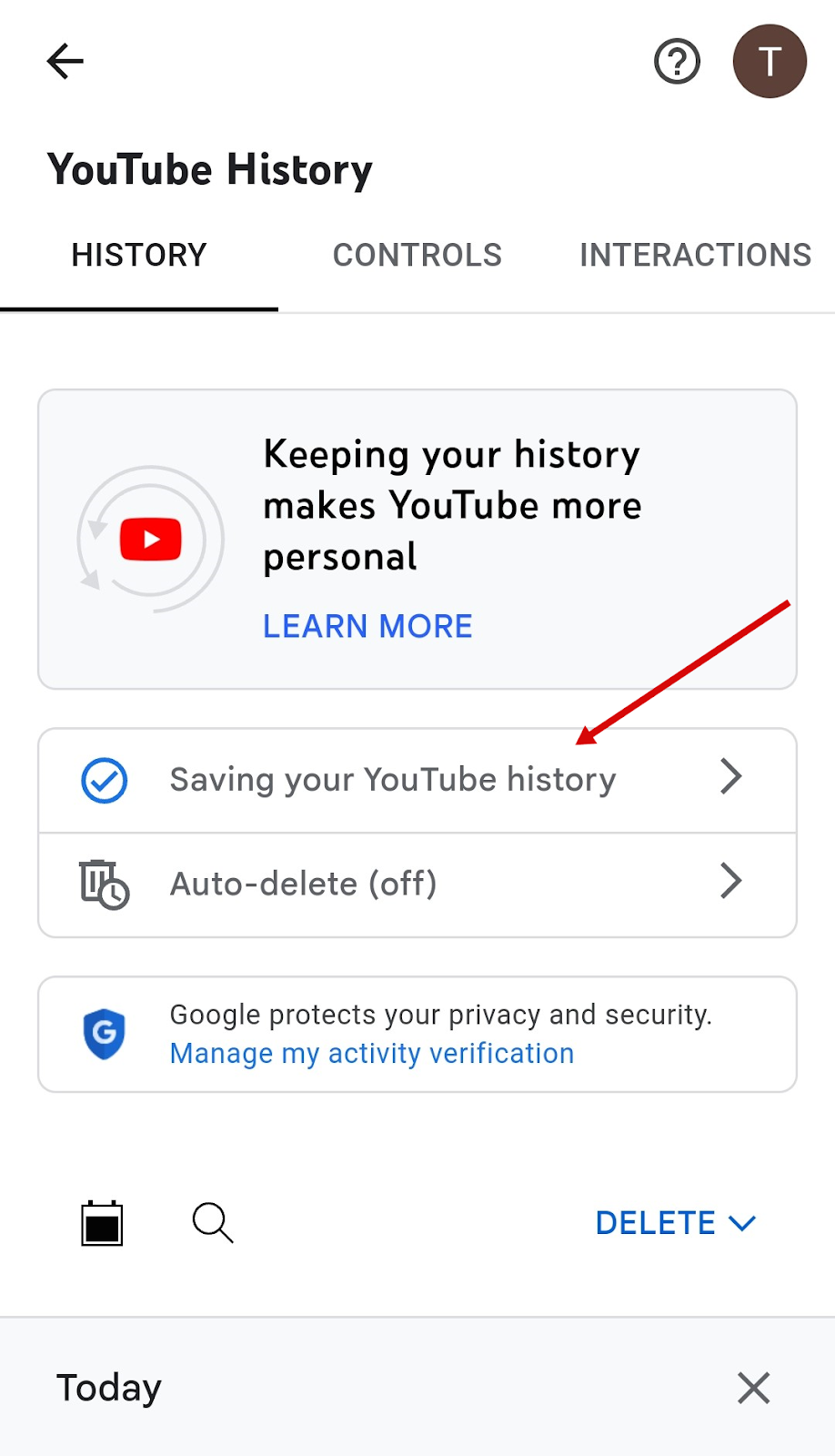The image displays a screenshot of a YouTube history page. In the top left corner, an arrow icon pointing to the left serves as a back button. On the top right, a question mark enclosed in a white circle with a brown outline is visible. The user profile section features a brown circle with a white letter 'T' in its center. Immediately below this, the text "YouTube History" is left-aligned in black font. Underneath this heading, there are three tabs: History, Controls, and Interactions, with the History tab currently selected. Further down, a prominent block of text encourages users to keep their history to make YouTube more personal, accompanied by a “Learn more” link and the YouTube logo on the left. There is a highlighted blue circle with a check mark and a red arrow pointing towards a section that emphasizes the importance of saving your YouTube history.